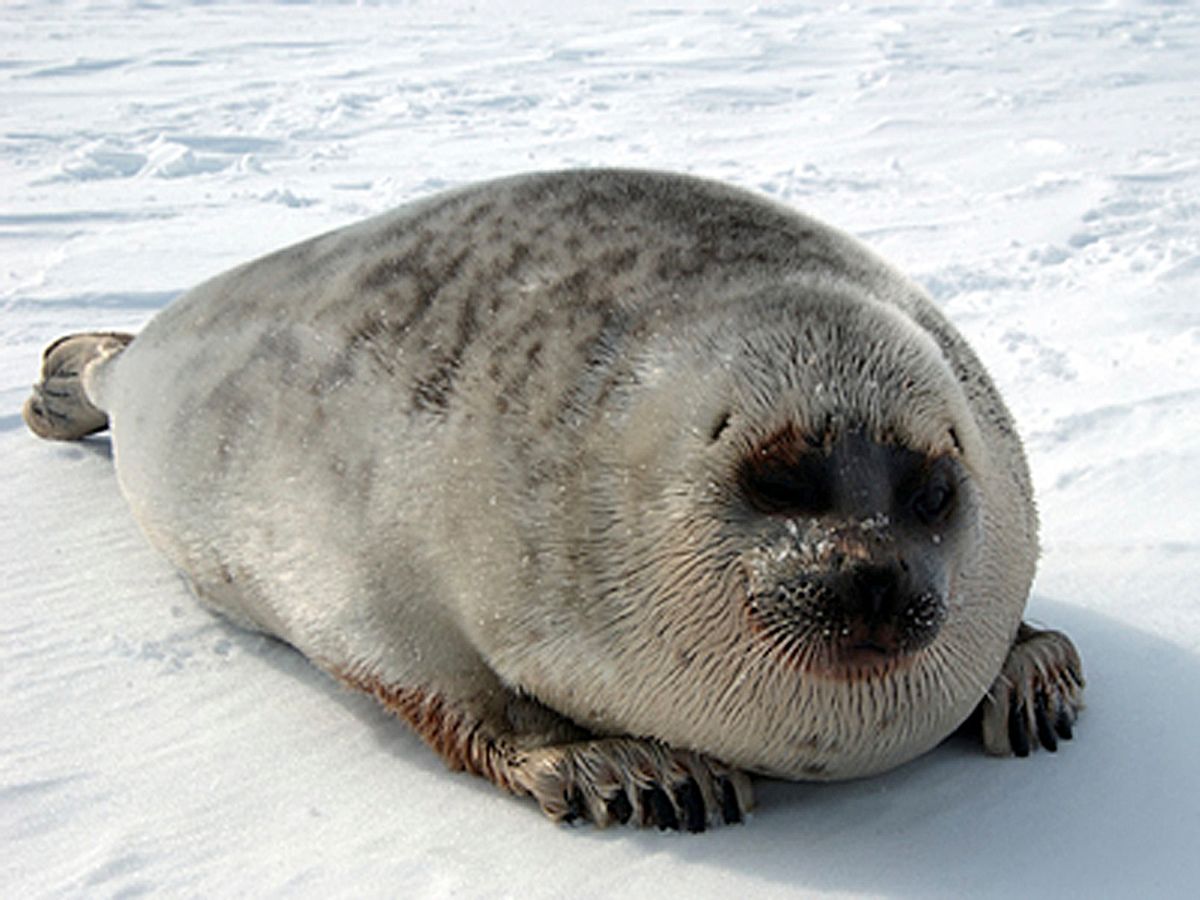This photograph showcases a very large seal, prominently positioned on a bright white snowy expanse in what appears to be an arctic or subarctic region. The seal, taking up most of the frame, is lying on its paws with its tail visible at the back, slightly to the left. Facing the camera, its head is tilted a bit to the right, revealing expressive black eyes surrounded by notable dark rings and a black snout, dusted with tiny flakes of snow. The seal's coat features a blend of lighter gray hues on the lower part, transitioning to darker gray and black speckles on the upper body, lending it a speckled appearance. The overall impression is of a pudgy, hefty creature, evidently well-adapted to its frigid environment with a substantial layer of insulating adipose tissue. The image, although of medium quality, offers considerable detail, though some finer features of the fur are slightly blurred. The entire background of the photograph is a pristine, undisturbed snowy landscape, captured in daylight, with no sky or additional elements visible.